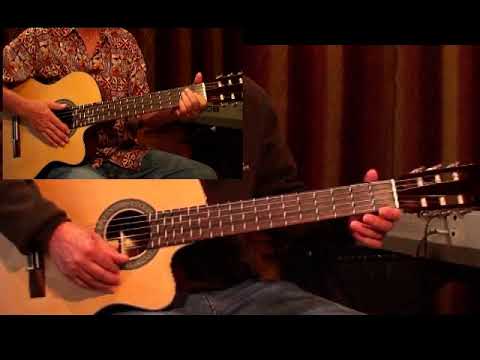The image depicts two individuals, each playing an acoustic guitar. Both persons are seated and wearing blue jeans, with their torsos, necks, and part of their legs visible, but their heads out of the frame. The larger figure in the foreground wears a brown button-up shirt with one button undone and strums the guitar with his right hand while holding the frets with his left hand. The background features a brown curtain behind him. Additionally, there's a guitar amplifier visible on the ground. Superimposed over this scene is a smaller, inset image of another person, who appears to be wearing a brown sweatshirt with a patterned design. This person also holds a wooden acoustic guitar, mirroring the strumming and fret-holding actions of the larger figure. The consistent brown curtain serves as the backdrop for both the larger and inset images, adding a sense of cohesion to the composition.